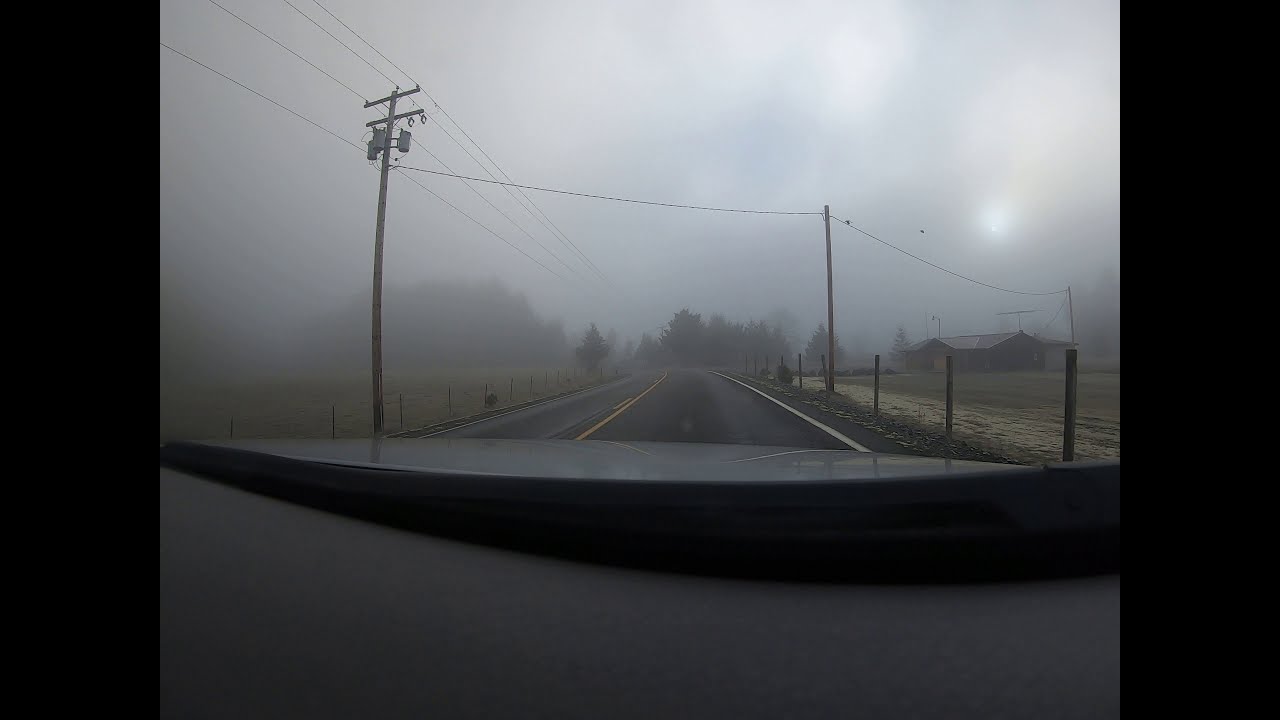This outdoor photo, likely taken from inside a car, captures a foggy, overcast day in a rural area. The image is dominated by a thick, pervasive gray fog, which obscures much of the scenery. The road, visible from the car’s dashboard at the bottom third of the frame, stretches ahead with a yellow center line and fields flanking both sides. Sparse trees are scattered along the roadside and in the distance. On the right side of the road, a house or possibly a barn is vaguely visible through the mist. Power lines extend across the scene, adding to the sense of an impending storm, whether it be a hurricane, tornado, or heavy rain with lightning. The image is framed by black borders on the left and right, enhancing the viewer's focus on the central, fog-laden vista.